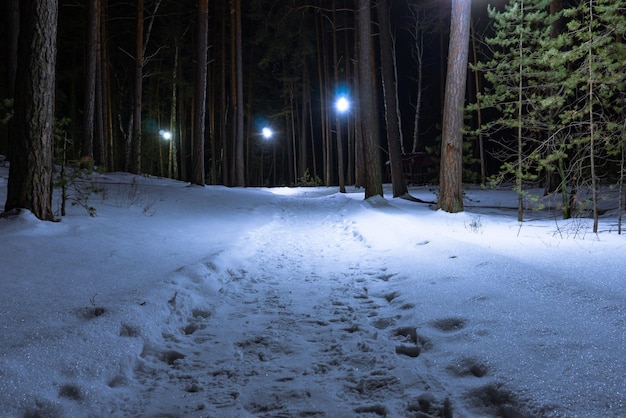The photograph captures a snowy path winding through a forest. The well-trodden trail, bordered by mounds of snow, stretches into the distance until it vanishes from sight. Numerous footprints mark the path, evidence of regular travel, causing the snow to compact in the center and build up along the edges. Tall trees, a mix of bare trunks and evergreen foliage, line both sides of the path. Wooden lampposts, emitting a soft white glow, illuminate the scene, casting bright patches on the snow and guiding the way forward. The sky above is pitch black, highlighting the nighttime setting and the stark contrast of the white, snow-covered landscape against the dark canopy. The ambient light from the lamps and the carefully cleared path suggest this is a well-maintained and frequently used route, likely transformed into a picturesque winter trail.